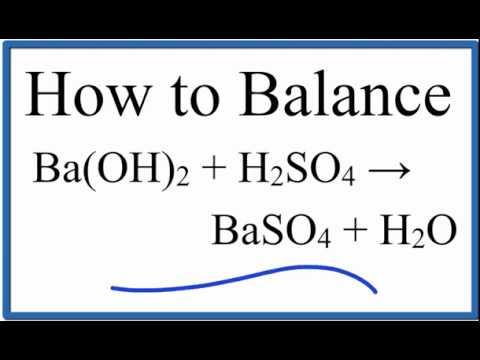The image is an illustration with a plain white rectangle bordered in blue, situated on a black background. Inside the rectangle, in bold black typeset, it says "How to Balance." Below this heading is a chemical equation: "Ba(OH)2 + H2SO4 → BaSO4 + H2O." The equation guides the viewer on how to balance the specified chemical formula. Beneath the typeset, there is a short, wavy blue line that spans from roughly the 25% mark to the 75% mark along the bottom of the white rectangle, resembling a wave in the ocean.